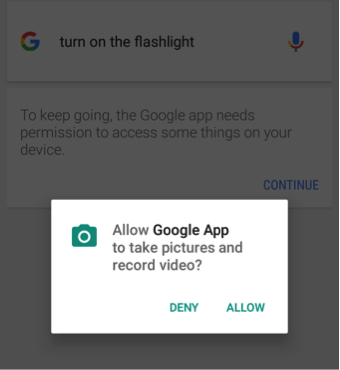The image displays a permission request page from the Google app. The background is a muted white, slightly grayed out due to an overlay box. The overlay box itself is predominantly white. At the top left of the box, there is a green camera icon. Adjacent to this icon, in black lettering, it says "Allow," followed by the bold black text, "Google app to take pictures and record video." 

Below this statement, there are two buttons in green text: "Deny" and "Allow." Beneath these options, the familiar "G" logo in rainbow colors is present, accompanied by the text "Turn on flashlight" on the same line, and a microphone icon appears next to it. 

A thin separator line runs across the box, and beneath it, a message reads: "To keep going, the Google app needs permission to access some things on your device." On the right side, just beneath this sentence, is the word "Continue" in blue letters.

This page is designed to request the user's permission for the Google app to access the device's camera and microphone functionalities. If the user denies the permission, the feature won't be activated. Allowing the permission will enable the app to function as intended, giving it access to the specified features.